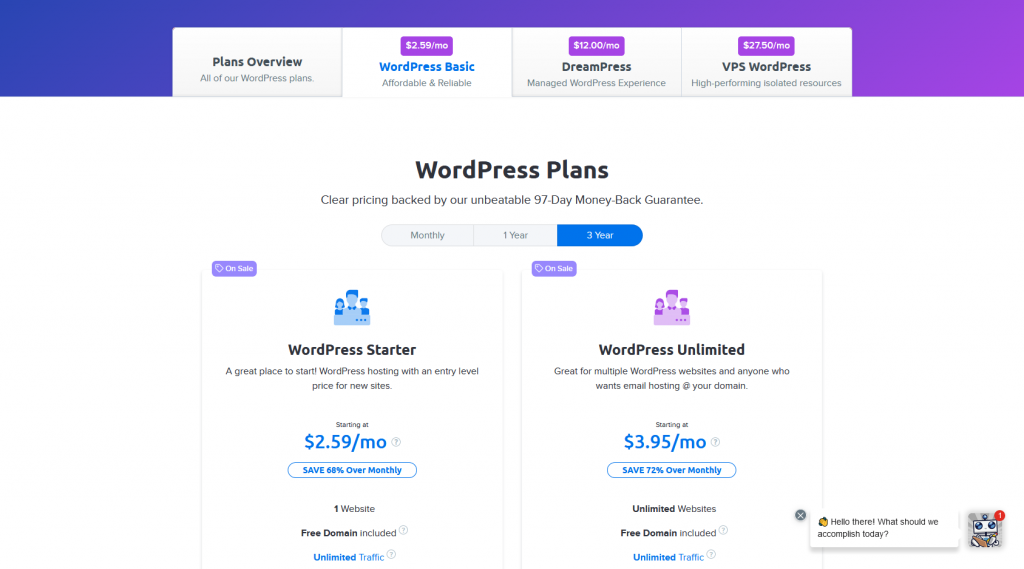The image features a WordPress website page with a prominent purple-toned banner located in the upper left-hand corner. The banner is two-shaded and has four centrally positioned selections: "Plans Overview," "WordPress Basic," "DreamPress," and "VPS WordPress." Three of these options display their prices, with "WordPress Basic" highlighted in a light sky blue color.

In the middle of the page, the text "WordPress Plans" is displayed, followed by the subtext, "Clear pricing backed by an unbeatable 97-day money-back guarantee." Below this section, there are options for "Monthly," "One Year," and "Three Year" pricing plans, with the "Three Year" option highlighted within an oval shape.

To the left side of the page, there is a section titled "WordPress Starter," marked with an icon that resembles a castle above it. The top left corner of this section features a purple oval or rectangular tag that reads "On Sale." Beneath the "Starter" heading, there's a centered paragraph detailing the plan, followed by its pricing information, which indicates a 68% savings over the monthly rate. This plan includes a certain number of websites and offers a free domain.

On the right side, there's another plan titled "WordPress Domain," which follows a similar format to the "Starter" plan. The pricing here is slightly higher, with one plan costing $2.59 and another $3.95. This section notes differences such as "Unlimited Websites" and additional features.

Overall, the page is designed to provide a clear and comprehensive overview of WordPress hosting plans, highlighting different pricing tiers, features, and promotional discounts to help users make an informed decision.